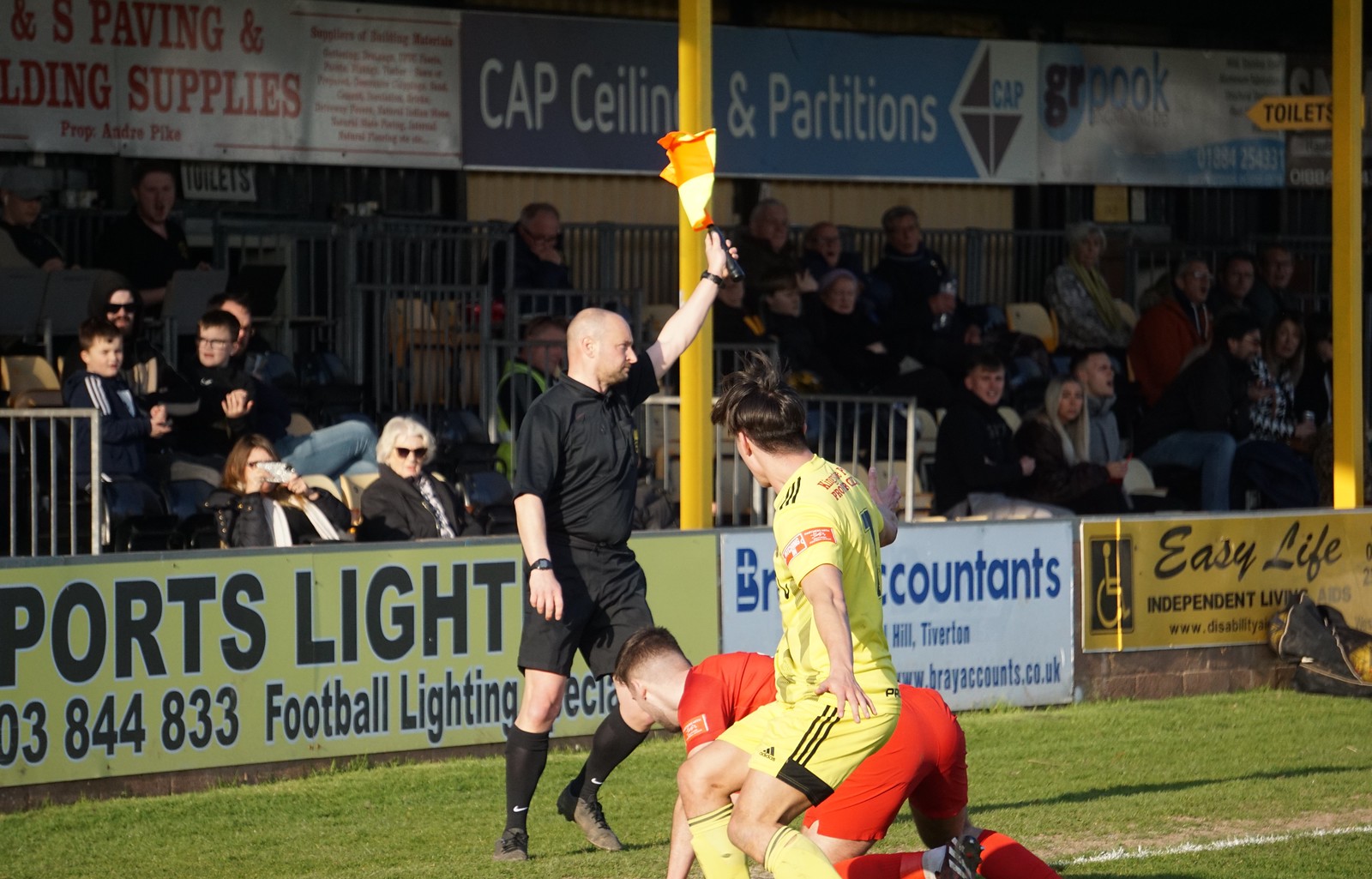In the vividly illuminated night-time setting of a soccer game, the image captures a dramatic moment on the field. At the center of the action, a man dressed in a black polo shirt and matching black soft pants stands authoritatively, holding aloft an orange and yellow flag, clearly identified as the referee. Directly in front of him, two players are engaged in a fierce contest. The player in the foreground, decked out in a complete yellow soccer uniform with yellow Adidas shorts, jersey, and socks, appears to be in the midst of maneuvering, arms outstretched as if to regain balance. Behind him, another player, clad in a red jersey, red shorts, and matching socks, is down on his hands and knees, seemingly recovering from a fall. Beyond the gripping on-field action, the spectator area in the background is densely packed, with no empty seats visible, and the crowds sitting in the dimly lit stands indicative of a well-attended evening match. Lining the area in front of the spectators are multiple advertisements, including ones for "Easy Life Independent Living Aids" and "Sports Light," offering a variety of products and services geared towards the sporting community. The overall ambiance, illuminated by the bright stadium lights, underscores the intensity and communal engagement of this nighttime soccer game.